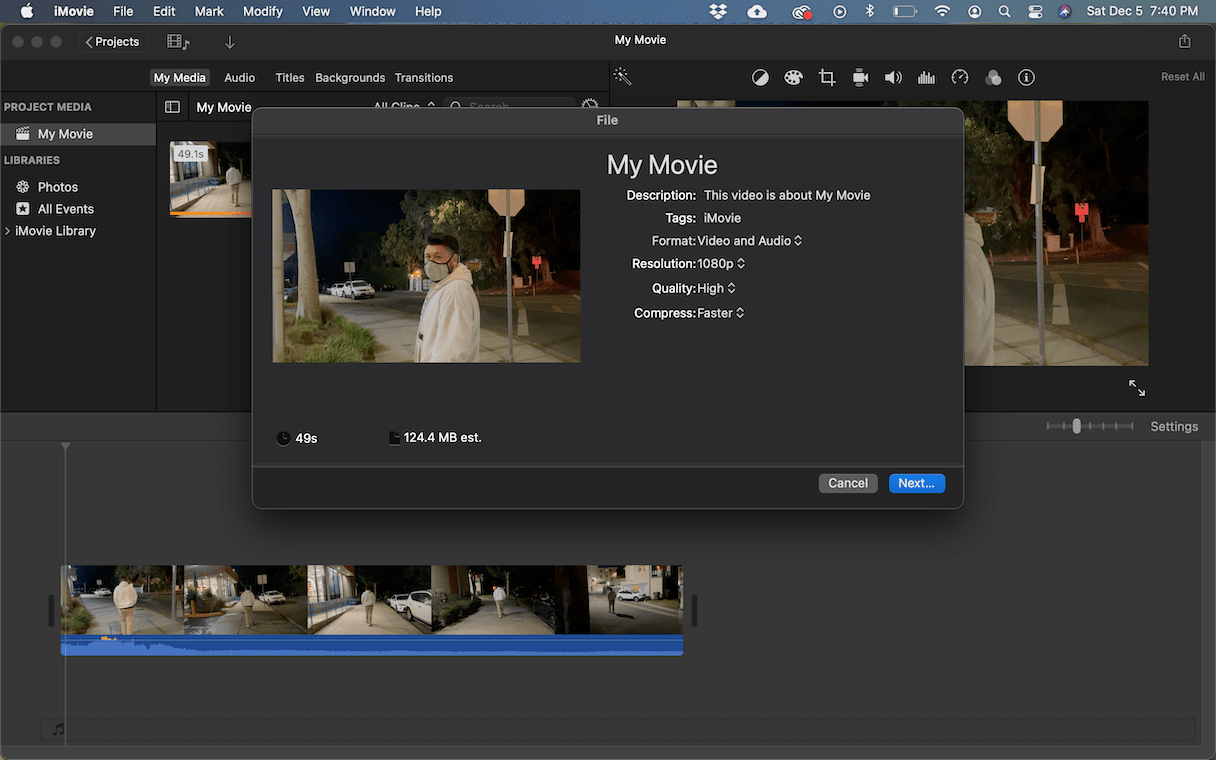Screenshot of iMovie Export Settings with Video Preview

In this detailed screenshot from iMovie's video editing software, the top-left corner prominently features the familiar Apple logo, followed by the application name "iMovie" and a series of menu options including File, Edit, Mark, Modify, View, Window, and Help. To the far right, the timestamp displays "7:40 PM" alongside the date "Saturday, December 5th."

The main focus of the image is a pop-up window for exporting a video titled "My Movie." The window provides multiple fields such as "Description," which reads "This video is about My Movie," and "Tags," which lists keywords like iMovie. The "Format" option is set to "Video and Audio," while the "Resolution" is specified as "1080p." The "Quality" is adjusted to "High," and "Compress" is set to "Faster."

At the bottom left corner of the pop-up, the video duration is noted as "49s," with an estimated file size of "124.4 MB." A preview frame is visible, showing a man wearing a mask standing on a sidewalk, providing a visual context to the video being exported.